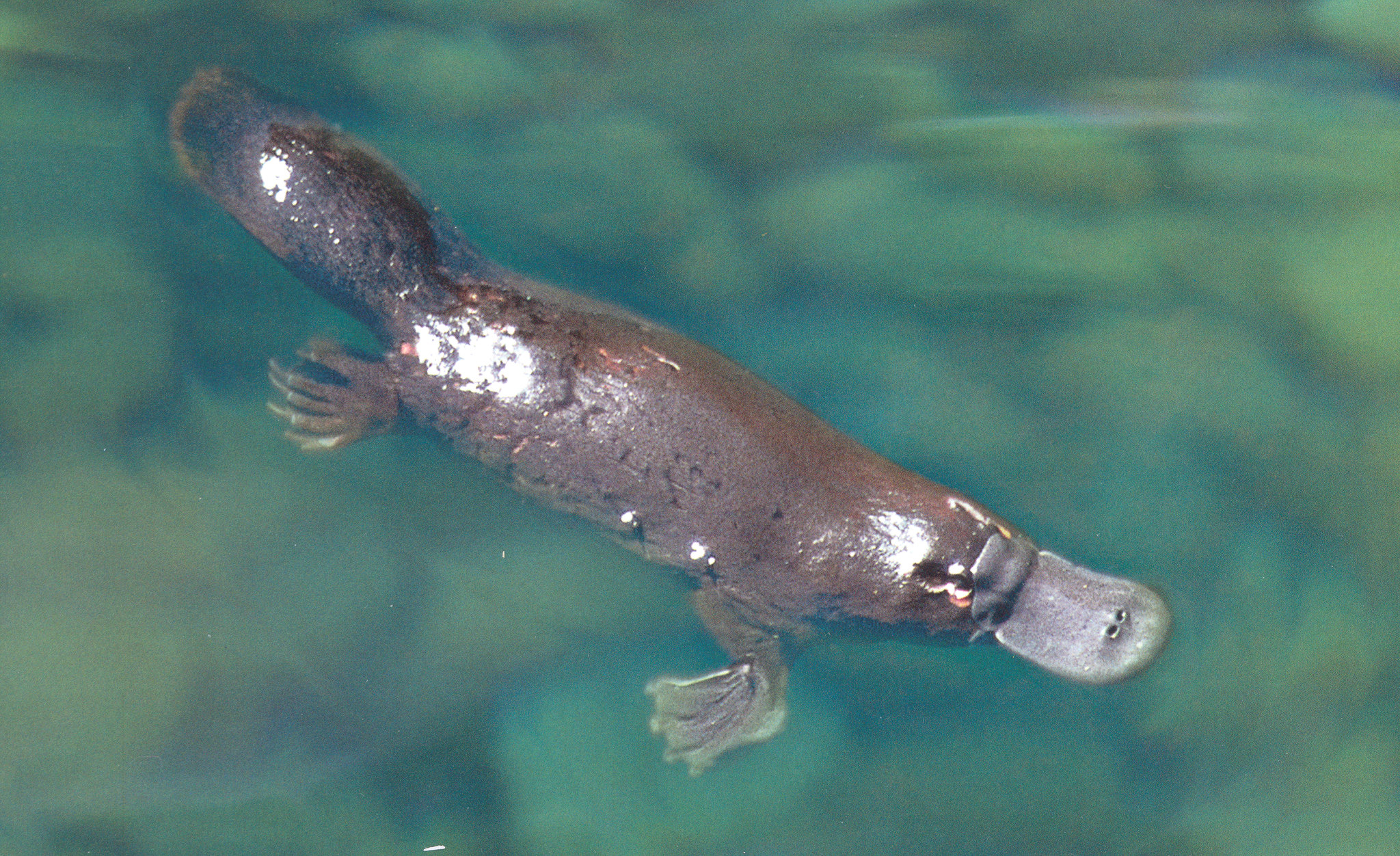The image captures an up-close, daytime scene of a baby platypus swimming diagonally through clear, greenish-blue water. You can see down into the water, which is interspersed with swirls of green and brown, likely effects of sunlight reflecting off plants or algae beneath the surface. The tiny creature is brown with a beaver-like tail that is about half the size of its body. It features a distinctive duckbill with noticeable nostrils on top, tiny eyes, and webbed feet; only two of these feet, the front and back left, are visible in the photo. The water's clarity reveals rocks and other elements at the bottom, enhancing the picture's natural appeal. There are no other elements or text in the image, emphasizing the serene, outdoor setting highlighted by glares of sunlight.